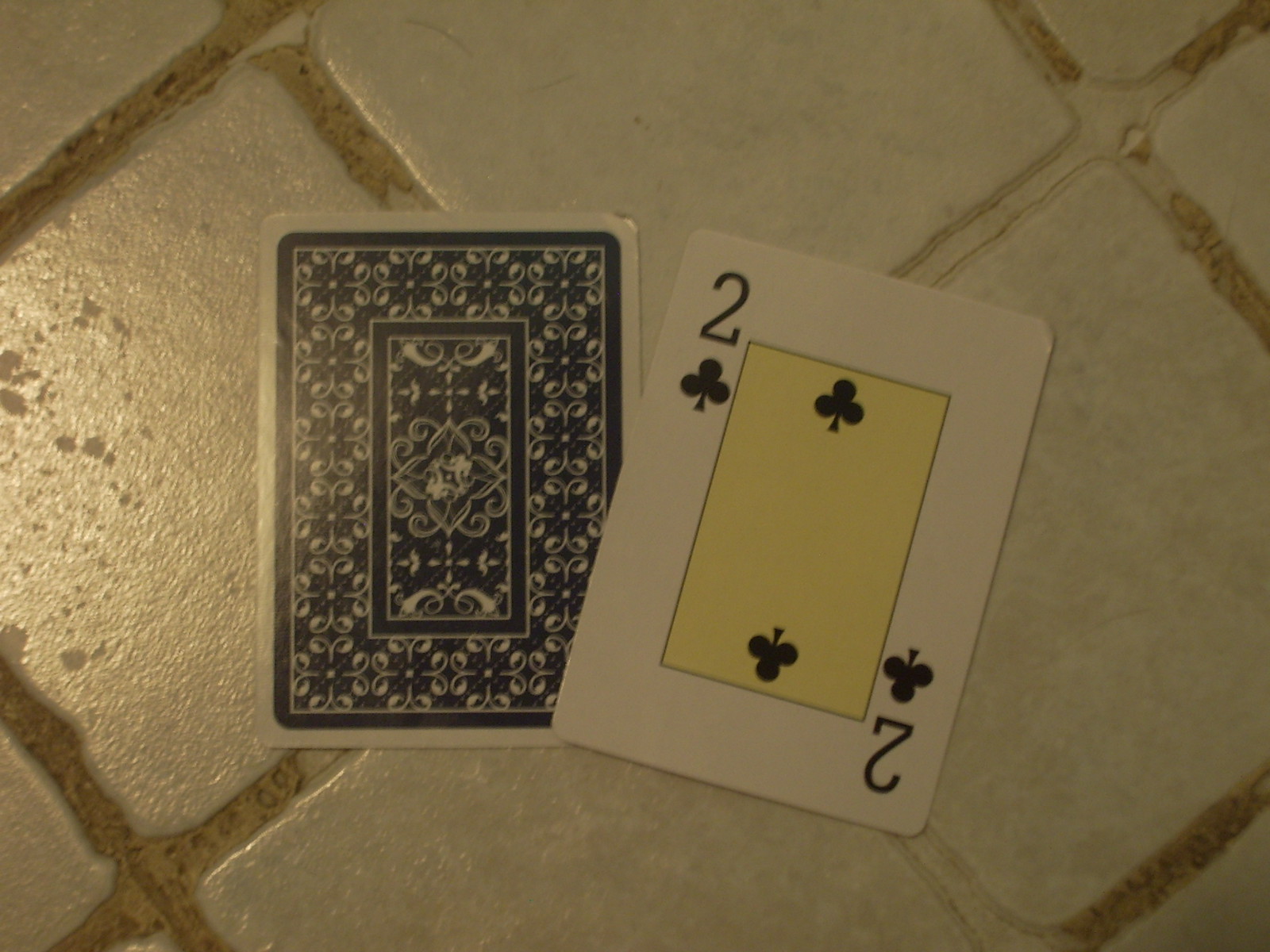In the center of this image, two playing cards are prominently featured, positioned side by side. The card on the left displays its back side, characterized by a dark blue color with an intricate flower-like design and bordered by a white frame. The card on the right reveals its front, identifying it as the Two of Clubs. This card features the number "2" in both the top left and bottom right corners, accompanied by black three-leaf clover symbols directly below each numeral and another centrally placed clover symbol. The card's background is a light yellow rectangular shape. Both cards exhibit signs of wear, with the upward-facing card showing a dense mark on its upper right-hand corner. The setting is a white tiled surface with light brown grout that shows fading in some areas, gradually blending to white.